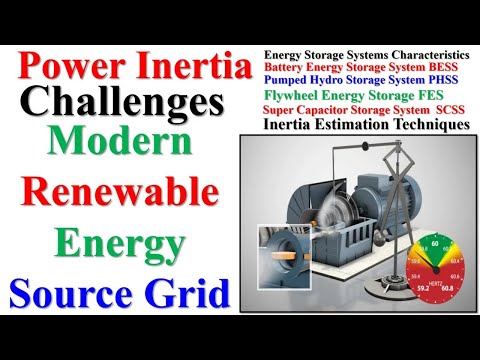The image appears to be an advertisement that seems to have been crafted using basic graphics software like Microsoft PowerPoint or Microsoft Paint, featuring rudimentary text and a picture. The left side of the image contains a list of words in various colors: "Power" in red, "Inertia" in black, "Challenges" in green, "Modern" in red, "Renewable" in green, "Energy" in blue, and "Source Grid" in distinct lines, each altering colors with each word.

On the right side, smaller text is more densely packed and describes various "Energy Storage Systems Characteristics." These include "Battery Energy Storage System (BESS)" in red, "Pumped Hydro Storage System (PHSS)" in blue, and "Supercapacitor Storage System (SCSS)" in red, followed by "Inertia Estimation Techniques" in black. The top and bottom edges of the image are cropped with black bars, indicating it might have been adjusted from a different aspect ratio.

Beneath this text is an image of what looks like a machine with a petrol blue color, featuring a turbine. The turbine has a rod connected to a stand on its right. In front of the turbine is a close-up of a portion of the machine, and to the bottom right is a gauge resembling a speedometer, labeled "Hertz," with sections marked in red, yellow, and green, indicating measurements around 59.2 to 60. The overall impression is that of a mechanical and technological focusing on modern renewable energy sources and storage solutions.